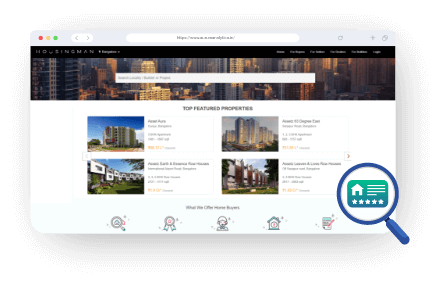The image depicts a website interface. At the top, there is a URL field set against a white background, though the resolution makes the URL unreadable. The browser's surrounding interface is silver, and no specific tab is highlighted. Below the URL field is a panoramic photograph featuring a skyline of numerous tall high-rises, bathed in the golden light typical of the "magic hour."

At the top of this photograph, a white search bar is visible, and while it contains black text, the content is not legible. Further down, the page consists of a white background featuring a section titled "TCP Featured Properties." This section showcases four property images, arranged in pairs with two images stacked vertically on either side. Each image has text next to it, though the specifics of the font remain unreadable.

In the bottom right corner, there is a prominent blue magnifying glass icon. Within this icon is a rectangular card that resembles a credit card, transitioning in color from blue at the bottom to green at the top. The card features five white stars at its base and includes an icon resembling a house, accompanied by several lines indicative of text or additional information.